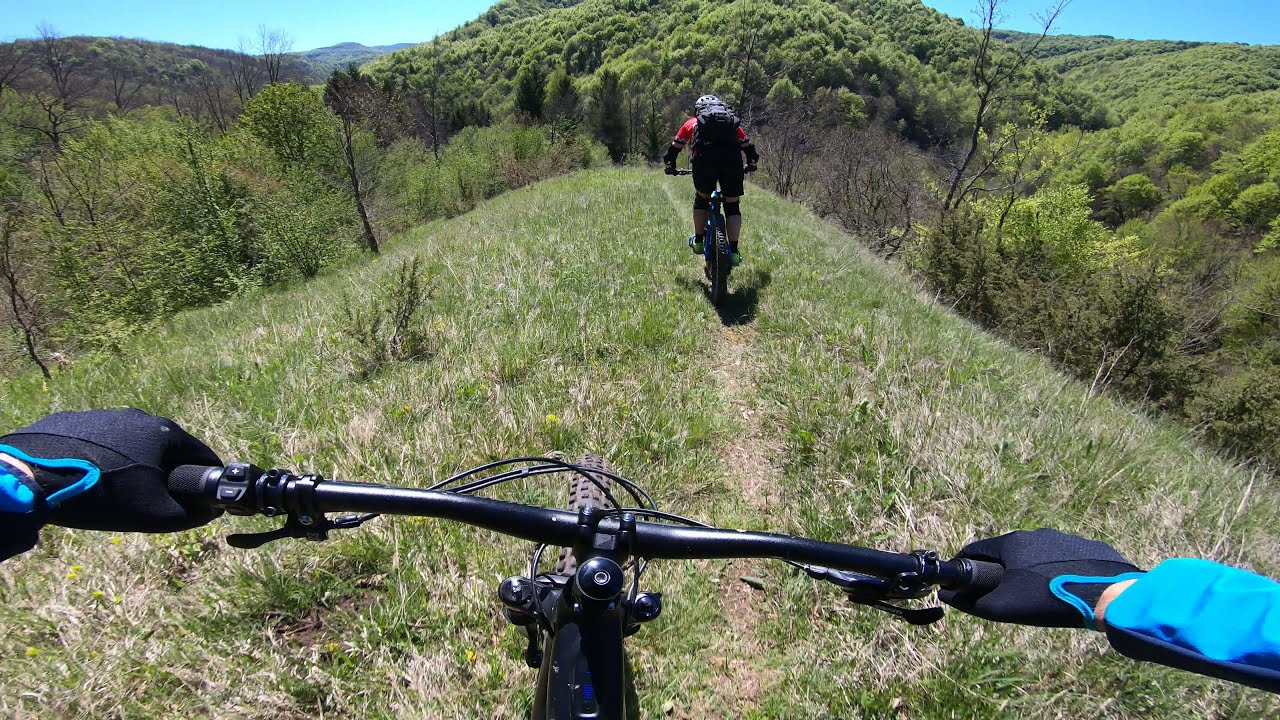Captured from a helmet camera, this vivid outdoor image shows two motorbike riders on a scenic mountain trail. The viewpoint is from the first rider, revealing his blue-sleeved arms and black gloves with blue trim gripping the handlebars of his mountain bike. He is descending a grassy hill along a faint, narrow path beneath a clear, bright blue sky. The grass appears dry with patches of dirt and dead grass interspersed throughout, suggesting late summer or early fall. Vegetation and lush trees surround the trail, which slopes down into a densely packed wooded valley ahead. In front of the vantage point, the second rider, wearing a red jacket and black backpack, is seen leaning forward on his bike, steering over the hill. The scene is framed by substantial hills reminiscent of the Appalachian range, enhancing the picturesque, forested landscape as both riders enjoy their sunny, mountainous adventure.